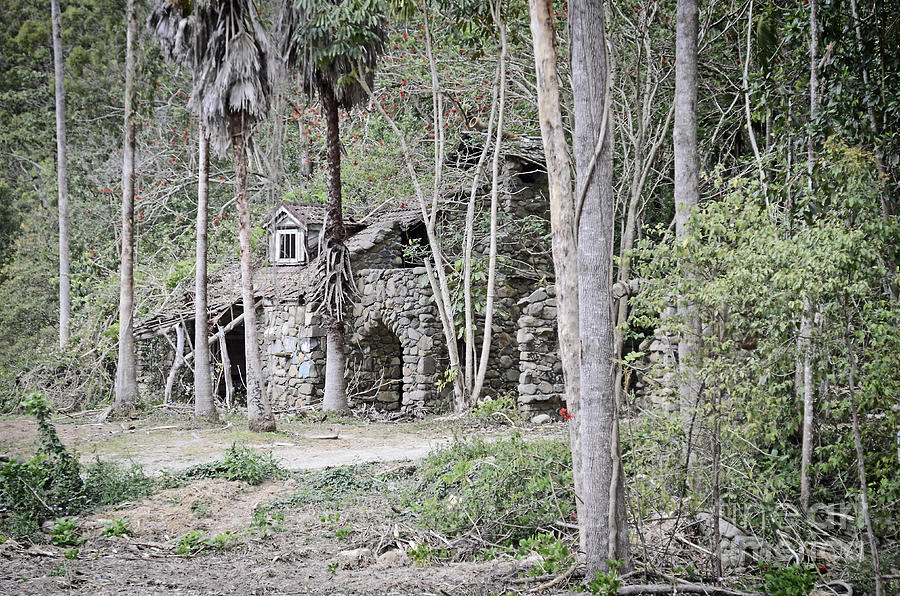This image depicts an old, stone house nestled within a dense, jungle-like forest dominated by palm trees and lush vegetation. The house's stone structure, held together with mortar, blends seamlessly with the wild backdrop, giving it an abandoned and timeless appearance. A single, upper window is visible on one of the rugged stone walls, reminiscent of a Cape Cod style. The roof appears to be constructed from twigs or straw, and tree branches from the surrounding forest extend over it, suggesting nature's reclamation of the area. The ground surrounding the house is covered in light-colored dirt or sand, devoid of grass, reinforcing its integration into the tropical environment. A narrow walkway can be seen leading into the forest on the right side, further enhancing the sense of mystery and exploration.